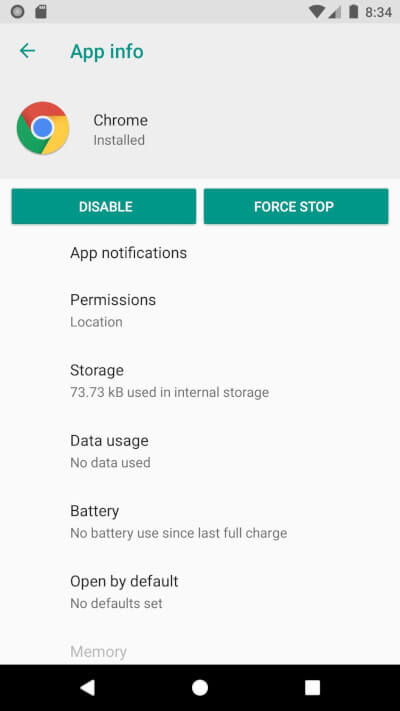The image is a mobile screenshot displaying the "App Info" page for Google Chrome. At the top, there's a gray status bar showing the time "8:34" in the top right corner, alongside fully charged battery and a gray SIM card icon. Below the status bar, the header section reads "App Info" in green text with a back arrow on the left. 

The main section showcases the Google Chrome logo, characterized by a blue circle surrounded by a red, yellow, and green swirl, beside the word "Chrome" followed by the status "Installed." Below this, there are two green rectangular buttons with white text: "Disable" on the left and "Force Stop" on the right. 

Further down, there are various details about the app: 
- **App notifications**
- **Permissions**
- **Location**
- **Storage**: 73.73 kilobytes used in internal storage
- **Data usage**: No data used
- **Battery**: No battery used since the last full charge
- **Open by default**: No default set
- **Memory**

At the bottom of the image, there's a thin black horizontal bar housing three white shapes: a left-pointing triangle on the left, a circle in the center, and a square on the right.